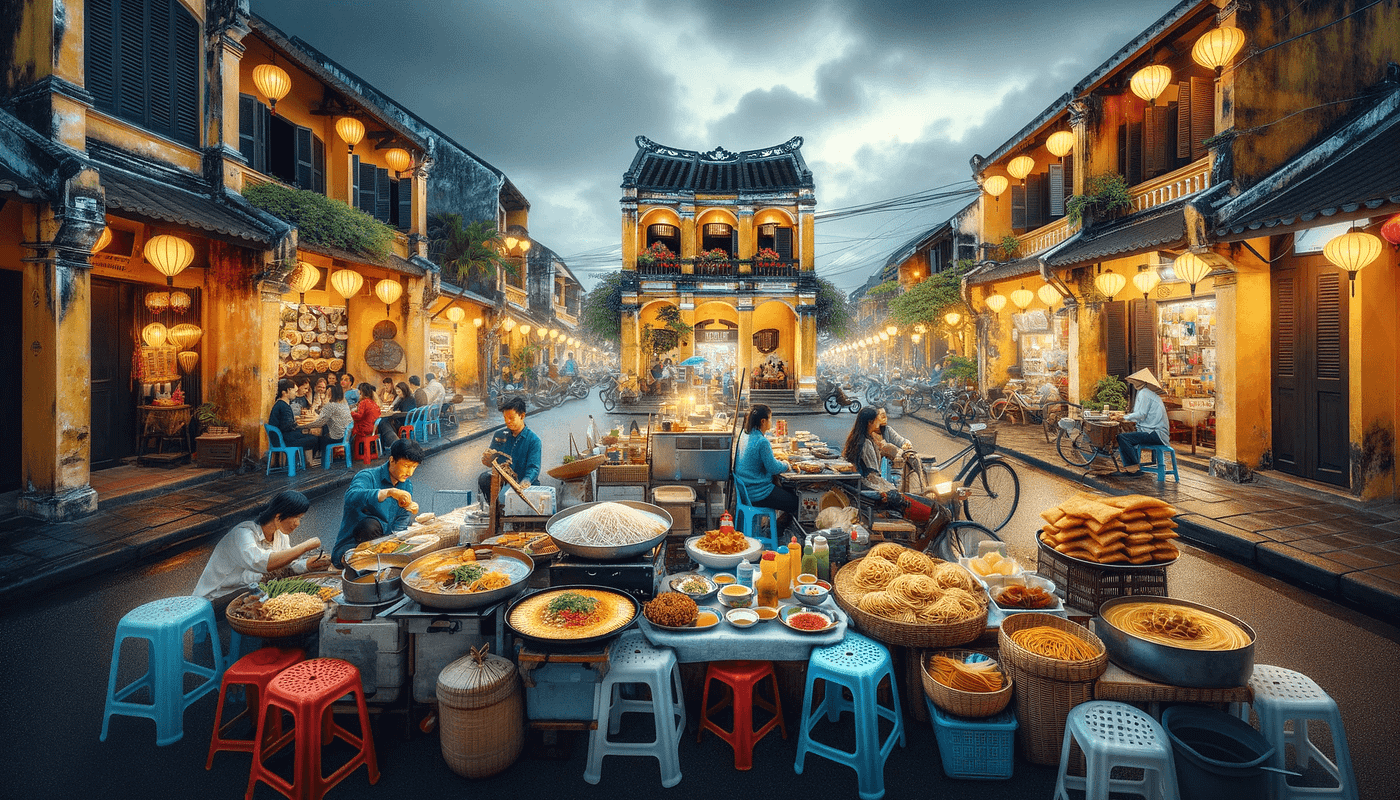This vibrant rectangular painting, approximately 6 inches wide and 3 inches high, vividly portrays a bustling night market scene set in an Asian street, possibly in China, Vietnam, or Korea. The viewer looks down at a street flanked by rows of yellow, two-story buildings adorned with brown doors and glowing amber-colored paper lanterns. The street is alive with activity, dominated by food vendors and dining patrons. 

In the center foreground, clusters of blue, red, and white plastic stools and low-lying tables are laden with large round plates and bowls brimming with various types of noodles. The noodles vary from dark yellow to light brown, thick and spirally to white and thin, accompanied by an assortment of condiments. To the left, vendors are seen preparing these dishes, and towards the back right, a lady is busily selling them. Scattered throughout the scene are people of Asian descent, some cooking, others dining on the sidewalks.

Bicycles are parked along both sides of the street, contributing to the dynamic energy of the market. In the distant background, a central two-story building stands with its upper level festooned with red flowers. The vivid array of blue and red colors in the clothing and stools, coupled with the warm glow of the lanterns, contrasts with the dark, cloudy night sky, enhancing the rich, atmospheric depth of this artistic rendition.